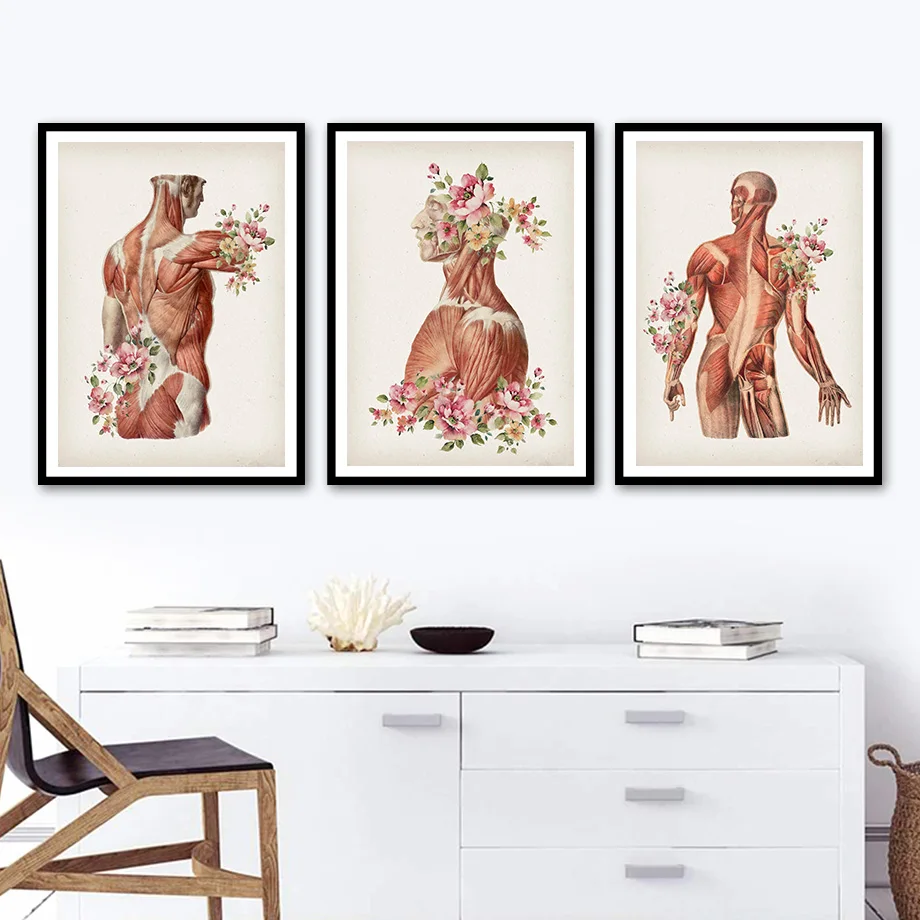The image features a minimalist, neatly arranged room dominated by a plain white dresser with silver drawer pulls. In the foreground, there is a wooden chair with a dark blue seat cushion, angled towards the 2 o'clock direction. On top of the dresser, there are two stacks of books, a small black bowl, and a quarter-visible basket on the right. Prominently displayed on the white wall behind the dresser are three black-framed anatomical drawings, evenly spaced. Each artwork showcases the human musculoskeletal system with detailed depictions of muscles, tendons, and ligaments. Notably, the drawings are adorned with pink and green floral motifs, resembling magnolia blossoms, sprouting from various parts of the body, one from the back and arm, another from the head and torso, and the last from the outstretched arms of a back view. The juxtaposition of human anatomy paired with the organic floral elements creates a striking and thought-provoking visual contrast.